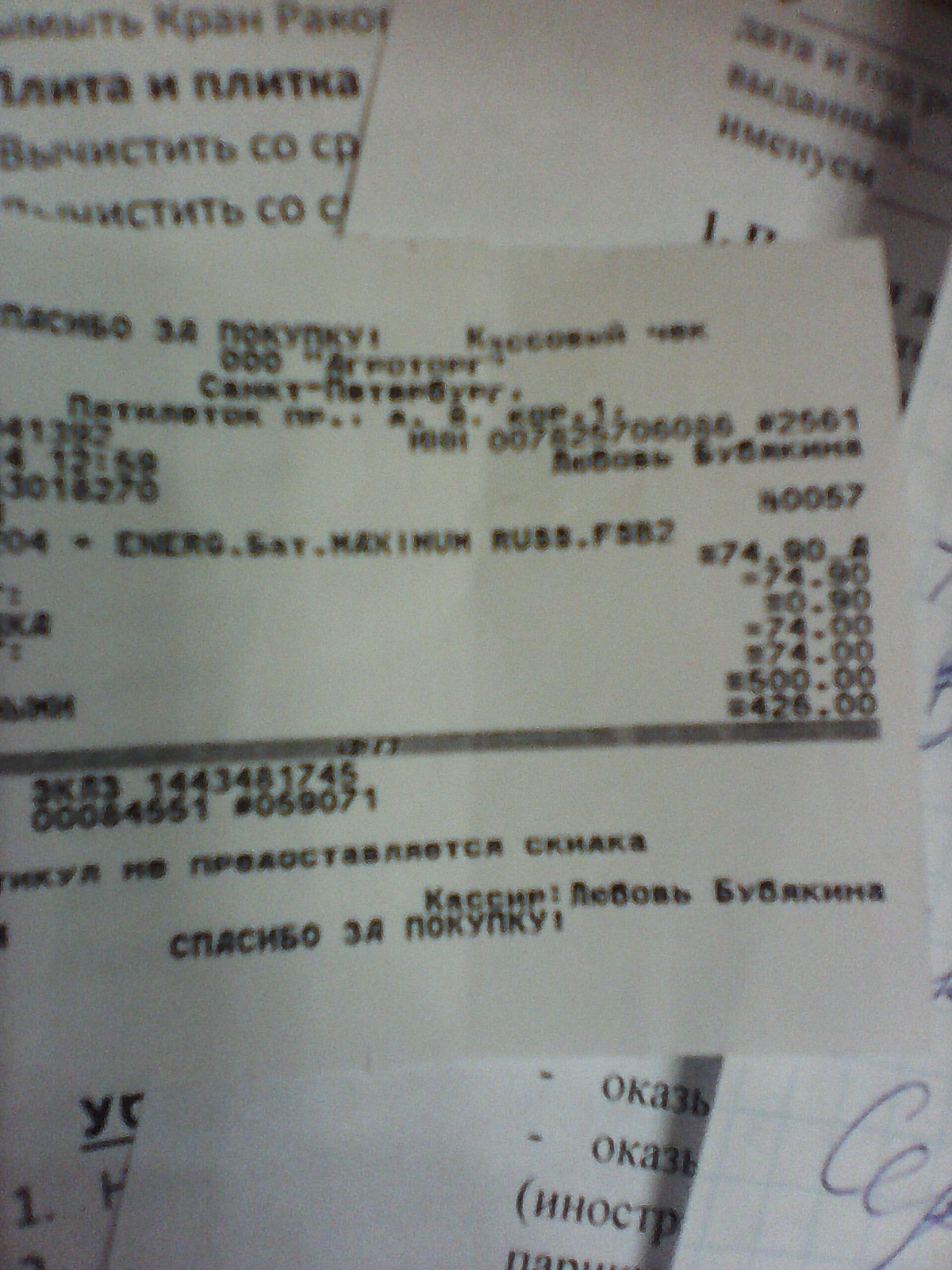This photograph captures a collection of assorted paperwork meticulously stacked on top of each other. The topmost sheet appears to be a receipt, which details multiple transactions with numbers such as 426, 574, and 7480 prominently visible. Although the exact language of the receipt is indiscernible, it bears a semblance to Middle Eastern or possibly Russian text. Beneath the receipt, there is a piece of paper covered in grids and handwritten notes in blue ink, suggesting perhaps a draft or some form of calculation. The bottom two layers consist of printed documents, characterized by black lettering on white paper, further contributing to the scholarly appearance of the ensemble. The overall setting of this image evokes a sense of meticulous record-keeping and organized chaos.